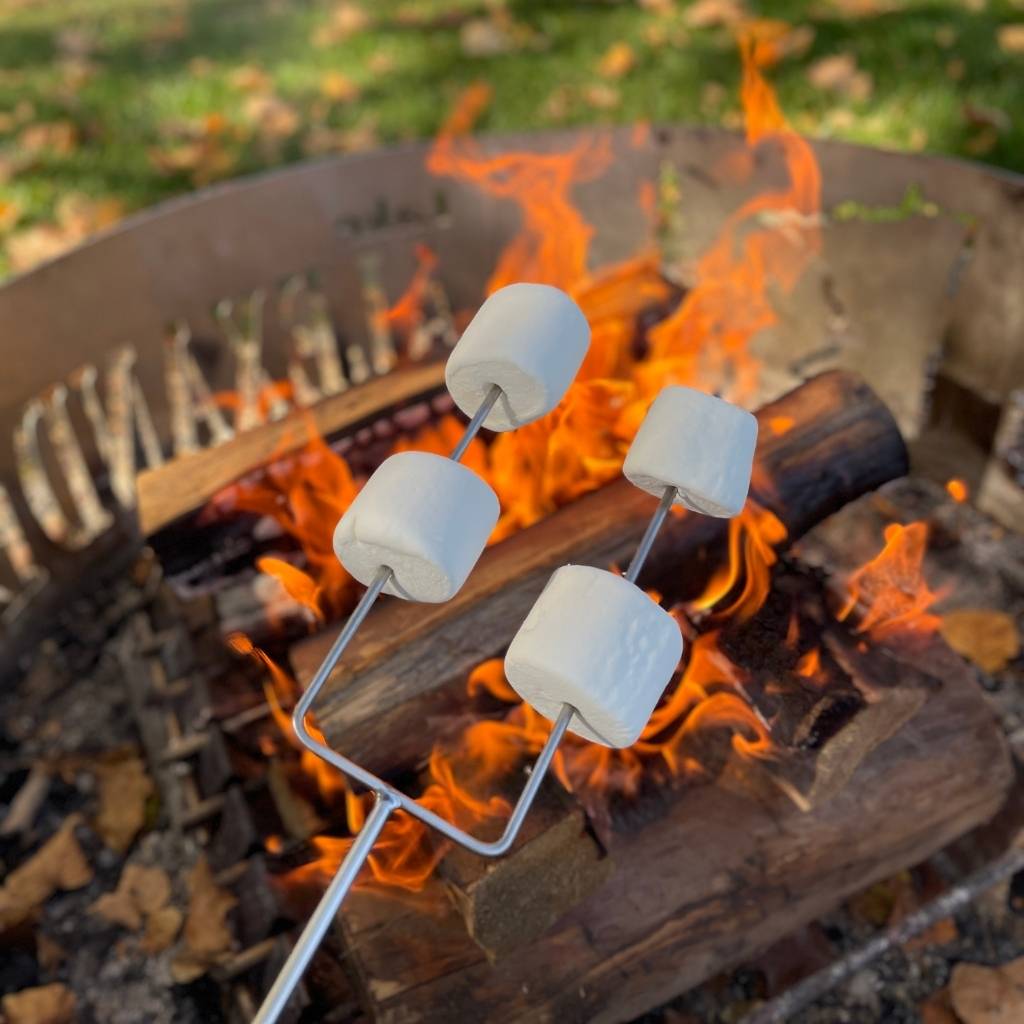In this photograph, a first-person view captures the outdoor setting during daylight, showing someone roasting four large fluffy white marshmallows on a silver skewer over a campfire. The skewer, which has a fork-like structure with two marshmallows on each prong, is held above an open flame in a metal fire pit, filled with stacked brown logs that are actively burning. The vivid orangish-red flames and glowing embers contrast with the surrounding green grass and scattered brown leaves visible in the background, emphasizing the sunny, outdoor campsite environment. Shadows of trees fall across the scene, and the image highlights the metal parts of the grill structure at the base of the fire pit, grounding the central focus on the marshmallows being perfectly toasted.